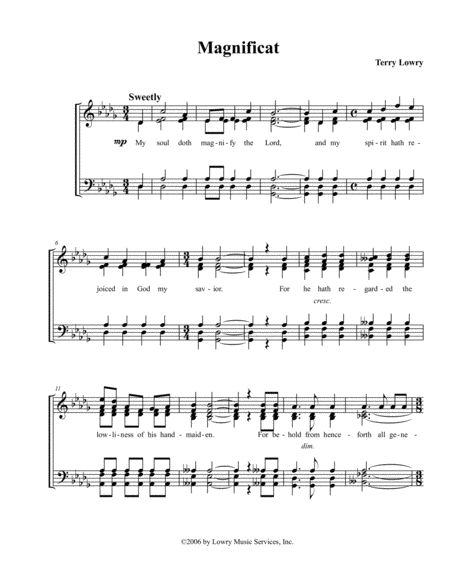The image features a scan of sheet music titled "Magnificat" by Terry Lowry. It displays a total of six bars, inclusive of both treble and bass clefs, suggesting it is likely the first page of this musical composition. The sheet music has a key signature of four flats, indicating it is in A flat major. At the top of the page, the tempo marking "Sweetly" is noted. The lyrics to the piece begin with "My soul doth magnify the Lord, and my spirit hath rejoiced in God my Savior." At the bottom, it shows a copyright notation, "© 2006 by Lowry Music Services, Inc." This sheet music is set against a white background and is a prominent example of church music notation.